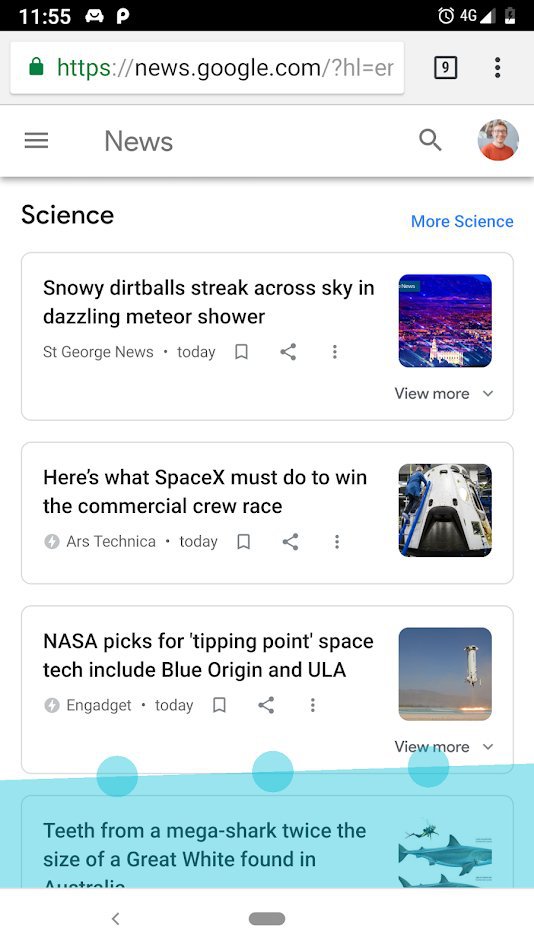This image is a screenshot taken from a smartphone displaying the Google News page. At the top, there's a black banner featuring the time "11:55," an icon of a car, the letter "P," and to the right, icons indicating a clock, 4G connectivity, and the cell phone signal and battery strength. Below the banner is the URL input bar showing "https://news.google.com?hl="er"." 

On a white background with black text, the header reads "News" and to the right is a circular profile image of a male with short, light-colored hair wearing a red shirt. Beneath the header, there are tabs labeled "Science" and "More Science," followed by rectangular sections designated for individual articles.

The top article is titled "Snowy dirt balls streak across sky in dazzling meteor shower" from St. George News, dated today. On the right side of this article, there's a brightly colored square photo showing an aerial view of a city. The next article is titled "Here's what SpaceX must do to win the Commercial Crew Race" from Ars Technica, dated today as well. Adjacent to this article, there's a square photo of a rocket's tip with a person climbing up the left side. Below that, another article is titled "NASA picks for tipping point space tech include Blue Origin and ULA" from Gadget, dated today. To the right of this article stands a square photo depicting a rocket in the process of taking off.